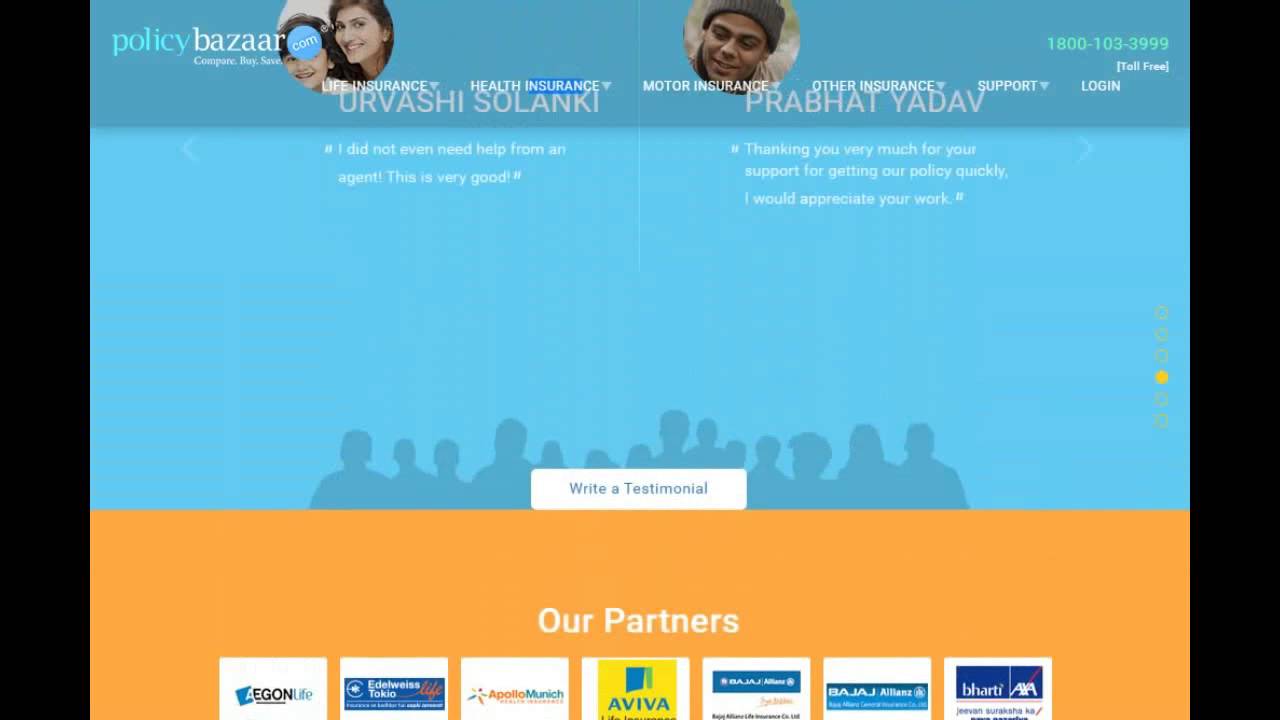The image features a promotional graphic for Policy Bazaar. The design is framed with black borders on the sides. The upper two-thirds of the central box is filled with a teal background, while the bottom third is in orange. 

At the top of the teal section, the text "Policy Bazaar" is prominently displayed, accompanied by the website URL "comparebigsave.com." Beneath this, categories like "Life Insurance," "Health Insurance," "Motor Insurance," and "Other Insurance" are listed. Additionally, options for "Support" and "Login" are mentioned.

In the teal segment, customer testimonials are showcased. Urvashi Solanki's testimonial reads, "I did not even need help from an agent, this is very good," followed by Prabhat Yadav's message of gratitude: "Thanking you very much for your support, for getting our policy quickly. I would appreciate your work." Silhouettes of people are seen at the bottom of the teal section, next to a white box prompting, "Write a testimonial."

The orange section highlights the company's partners, listing "AN Life, Edelweiss Tokyo Life, Apollo Munich, Aviva, Bajaj Allianz, and Bharti."

Overall, the graphic efficiently communicates the service offerings and client satisfaction associated with Policy Bazaar, while also showcasing its trusted partners.